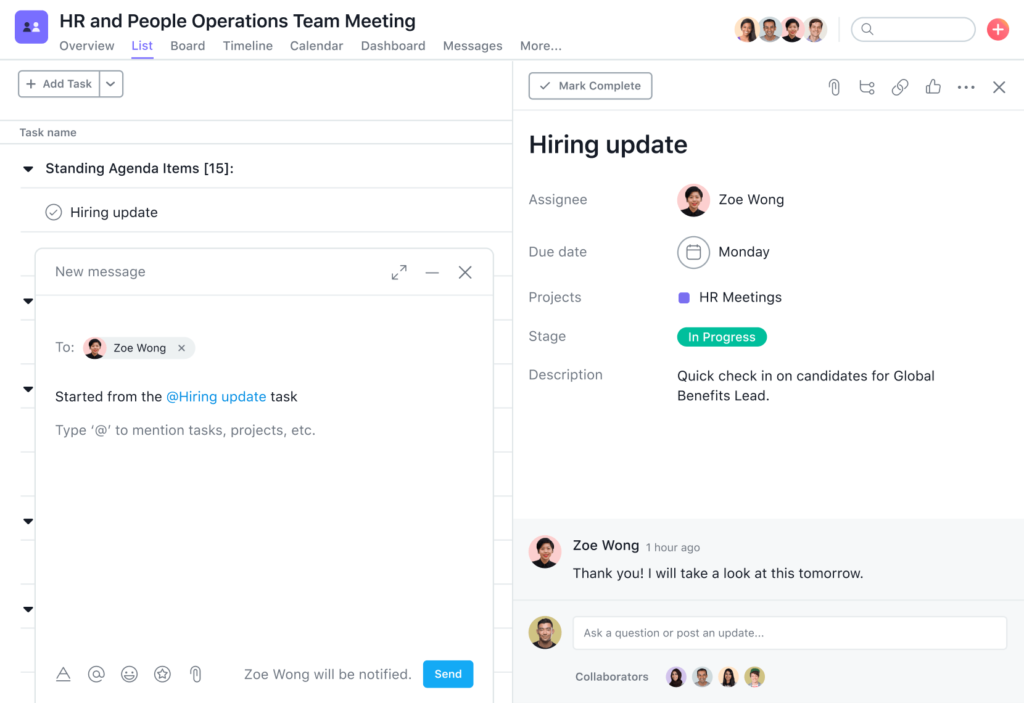This is an interface designed for managing team meetings online. In the top left corner, there's a blue square with rounded corners, featuring a small black and white icon depicting two people. Next to the icon, a title reads "HR and People Operations Team Meeting." Below the title, a navigation menu includes options such as Overview, List, Board, Timeline, Calendar, Dashboard, Messages, and more (indicated by three dots). The List section is highlighted in blue and underlined, indicating that the content displayed is from this section.

In the upper right corner, there are four user profile pictures arranged in circles, a search bar, and a plus button. The main content area on the left side includes a section for adding tasks, featuring fields for task names and a drop-down menu titled "Standing Agenda Items (15)." It also includes a hiring update and options for team members to add messages related to specific tasks.

On the right side, the interface provides additional functionalities for each task, including options to mark tasks as complete, assign them to individuals, set due dates, specify the related project, and check the current stage. There are also fields for detailed descriptions and sections for team members to leave comments.